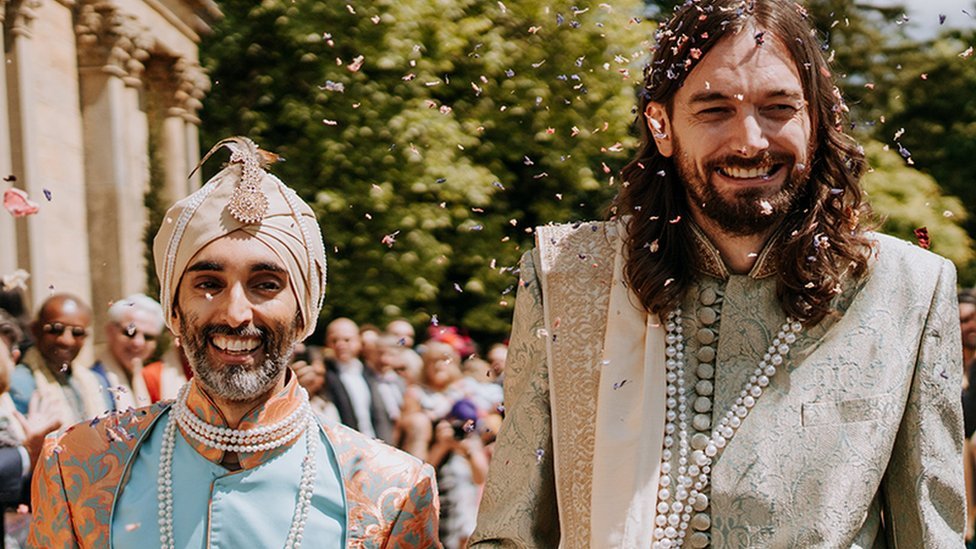The image captures two men walking towards the camera amidst a celebratory atmosphere with confetti swirling around them. The man on the left, notably shorter, wears an intricately embroidered peach and baby blue suit paired with a blue vest. His attire is complemented by a distinctive ivory turban adorned with a gold ornament. His salt-and-pepper beard adds a touch of maturity to his appearance, and long strands of pearls drape gracefully around his neck and chest. Beside him, the taller man sports a traditional silk suit in green and beige, fastened with looped buttons. This man, with fair skin, has long, flowing curly hair extending below his shoulders, accompanied by a well-groomed brown beard and mustache. He, too, wears an elegant chain of pearls. Both men are beaming with joy, suggesting the significance of the occasion. In the background, a captivated crowd watches intently, some wearing sunglasses due to the bright sunny day. The setting features big trees and a temple-like structure on the left, further enhancing the festive ambiance. This scene likely depicts a celebratory or ceremonial event, possibly a wedding, given the elaborate attire and the joyous expressions on their faces.